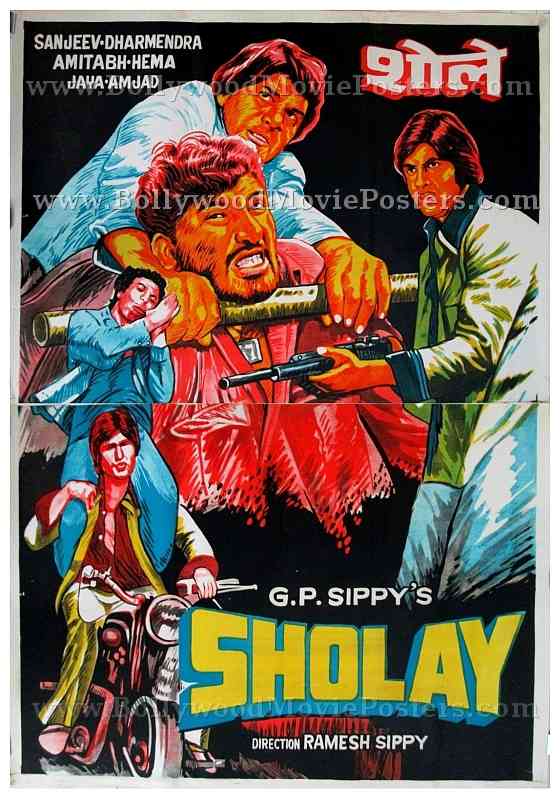This detailed vintage movie poster has a striking, cartoon-stylized design set against a black background and a watermark reading "www.BollywoodMoviePosters.com". In the bottom right-hand corner, yellow text on a blue background says "Cholet." Above this, it features "G.P. Sippies" in white font, and below it reads "Director Ramesh Sippy." 

In the foreground, to the bottom left, a man in a green jacket rides a motorcycle with another man in a blue suit resting on his shoulders in a prayer-like, sleeping position. Dominating the top left, a man with orange-toned skin, dark hair, and a red suit is being choked with a large cylinder tube by another man in a light blue shirt. To the right side, another figure in a green shirt and blue pants points a gun. All characters are rendered in a dynamic cartoon style that evokes the vibrant, action-packed feel of a classic Indian movie poster.